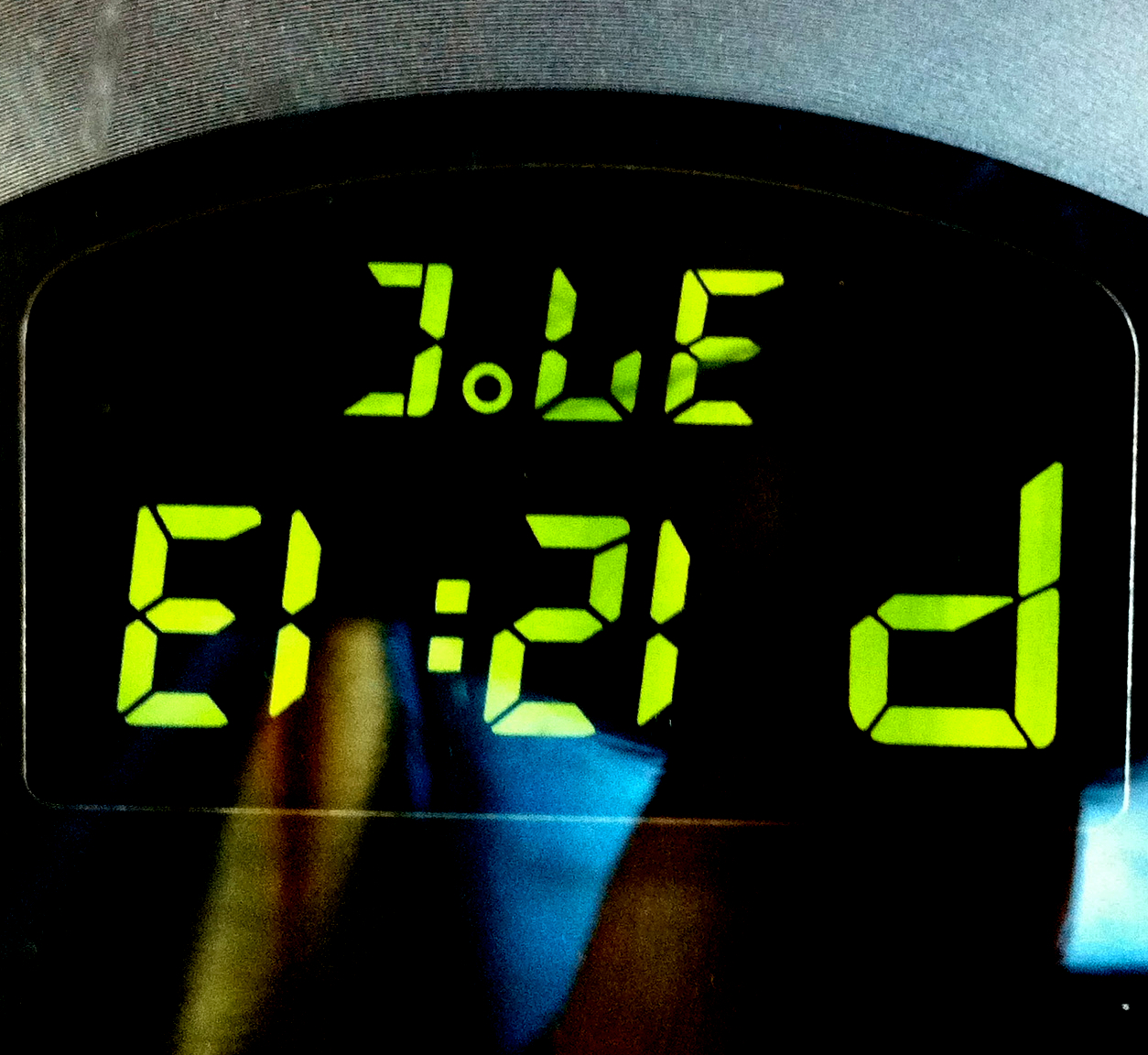In this intriguing image, a black digital clock with rounded edges, lying against a backdrop of blue jeans, takes the spotlight. The digital display on the clock, mirrored and upside down, reveals the time as "P12:13" and the temperature as "37°C." The reflection on the clock's surface faintly captures the image of an arm and a table, as well as a hint of something blue, adding an extra layer of depth to this everyday scene.